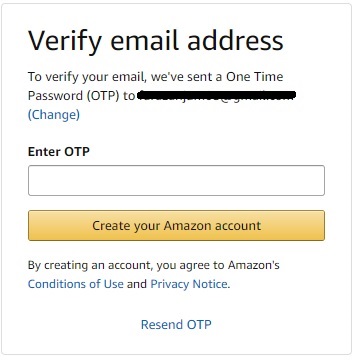This image is a screenshot of an Amazon verification pop-up box. The pop-up features a white square with a pale grey outline. At the top-left corner, there is a large, bold text that reads "Verify Email Address." Below this, a space separates it from the smaller text that reads, "To verify your email, we've sent a one-time password (OTP) to [email address redacted]." Directly underneath, there is a blue hyperlink labeled "Change," which allows users to alter the provided email address.

Following this, the text "Enter OTP" appears in bold, black font, next to an empty white text box where the user is expected to input the OTP they have received. Below this input field is a goldish yellow button labeled "Create your Amazon account," which is identical in size to the OTP input field.

At the bottom of the pop-up, there is a disclaimer that reads, "By creating an account, you agree to Amazon's Conditions of Use and Privacy Notice," with "Conditions of Use" and "Privacy Notice" in blue, indicating they are clickable links. Centered at the very bottom, it says "Resend OTP."